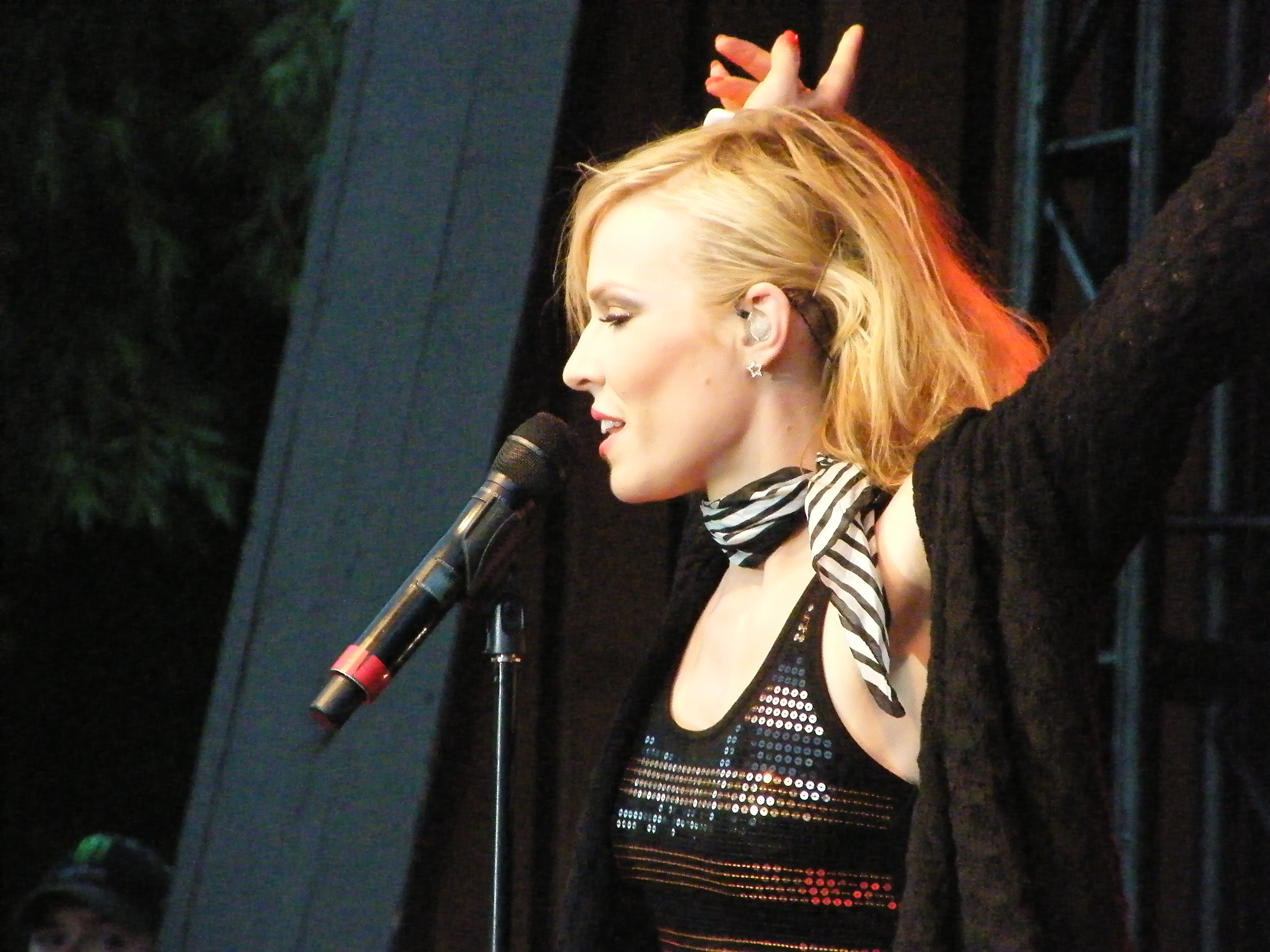This image captures a blonde woman with fair skin, her shoulder-length hair styled in a slightly messy, side-parted fashion, partially covering her face. She is adorned with eye makeup and blush. Her attire includes a black, sequined tank top beneath a long black sweater, complemented by a black and white striped scarf tied around her neck. 

The woman is centrally positioned in the frame, shown from the chest up, with both arms raised high and slightly behind her. She is singing, her mouth partially open and eyes partially closed, into a black and red microphone held by a black stand situated to her left. Additionally, she has an earpiece in her ear.

The background features a tall, predominantly black wall with hints of navy blue, suggesting the setting is a stage, likely filled with various black equipment or tall metal structures. The image is devoid of any text, focusing solely on the woman's expressive performance.